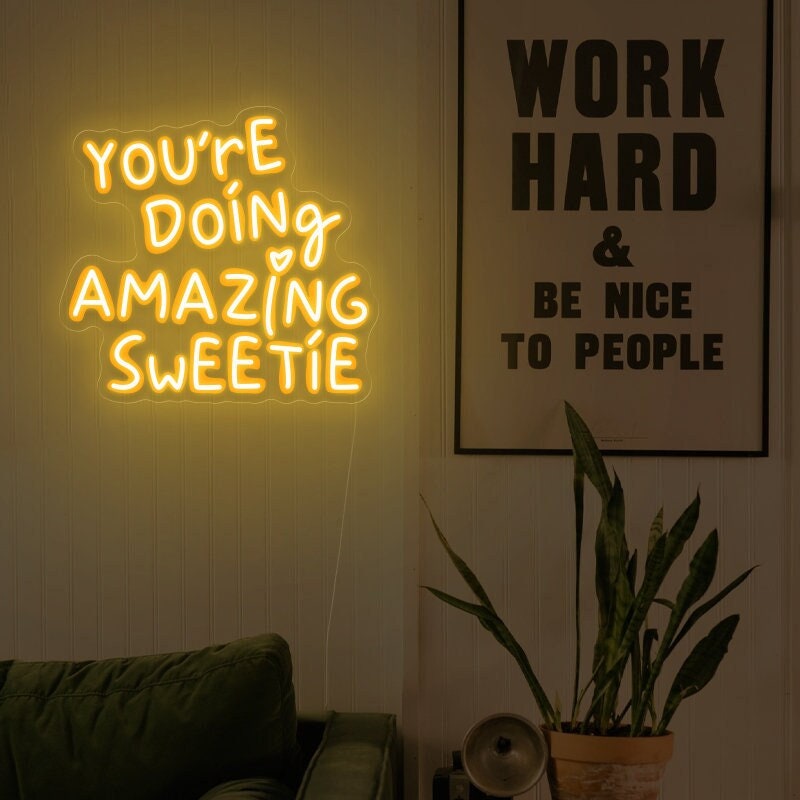The photograph depicts a cozy and stylish living room with a white wall featuring vertical indentations. Prominently displayed on the left side of the wall is a glowing yellow neon sign that reads, "You're doing amazing, sweetie." This sign is positioned above a green sofa. To its right, a framed poster with a black border and large block letters on a cream background states, "Work hard and be nice to people." A cord from the neon sign runs down the wall. In front of the poster, a tall potted snake plant stretches up, housed in a standard brown ceramic pot. The clean and inviting room also includes another potted plant, contributing to the room's welcoming atmosphere.